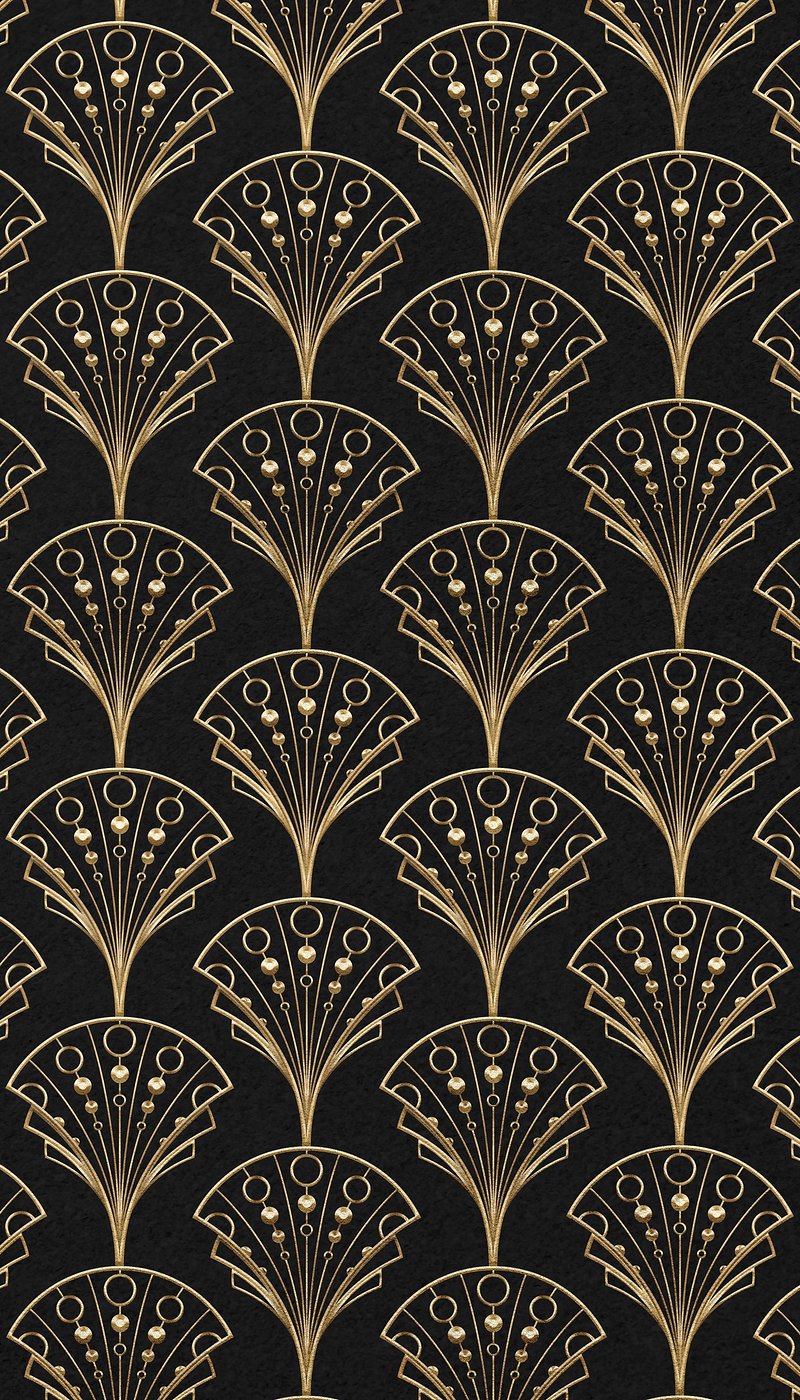This illustration, resembling a highly ornate wallpaper pattern, features a series of intricately designed, fan-shaped objects arranged in a grid-like structure against a stark black background. Executed in varying shades of very light brown, beige, and gold, the fans display a distinctly Art Deco style with intricate detailing. Each fan element is layered with delicate brown lines and accented interiors, featuring a series of rounded circles near the top. Closer examination reveals a tiered structure with five hollow black circles at the highest point, followed by three, and then two solid brown circles, completing the pattern as it inaugurates from a pointy base. The repetition of these fan motifs—organized in alternating columns of five and six—creates a cohesive and aesthetically appealing design. The entire composition is visually rich yet uniform, dominated exclusively by the shades of beige, tan, and black, enhancing its suitability and aesthetic appeal for wallpaper or wrapping paper.